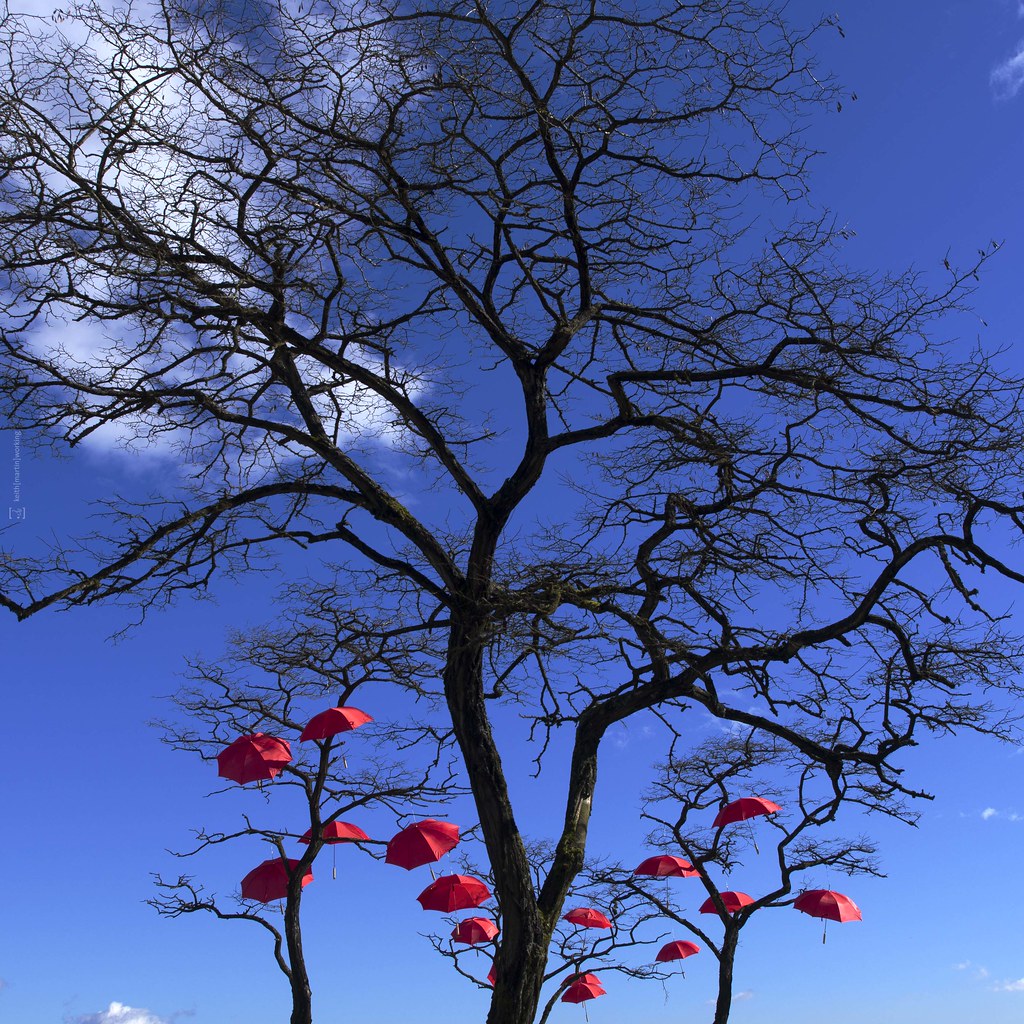In this color photograph with a square orientation, the vantage point directs us upward towards a richly deep blue sky that gracefully lightens towards the horizon. Dominating the scene is a large, leafless tree standing prominently in the center of the frame. Its trunk branches out expansively to the left and right, with a myriad of intricate branches weaving through almost the entirety of the image. To the left of the large tree, there is a prominent patch of white clouds. Surrounding the central tree, there are a couple of smaller, more slender trees in the background, which appear relatively smaller, perhaps due to their distance. Throughout the branches of all the trees, numerous open red umbrellas are distinctly visible, captured from various angles and lightly contrasting against the otherwise natural setting. The fine handles of the umbrellas are faintly discernible, adding an element of intrigue. The photograph leaves an open question as to whether these vibrant umbrellas have been artfully placed in real life, suggesting an artistic installation, or if they were superimposed digitally as part of a creative edit. This juxtaposition of natural and artificial elements adds depth and curiosity to the composition.